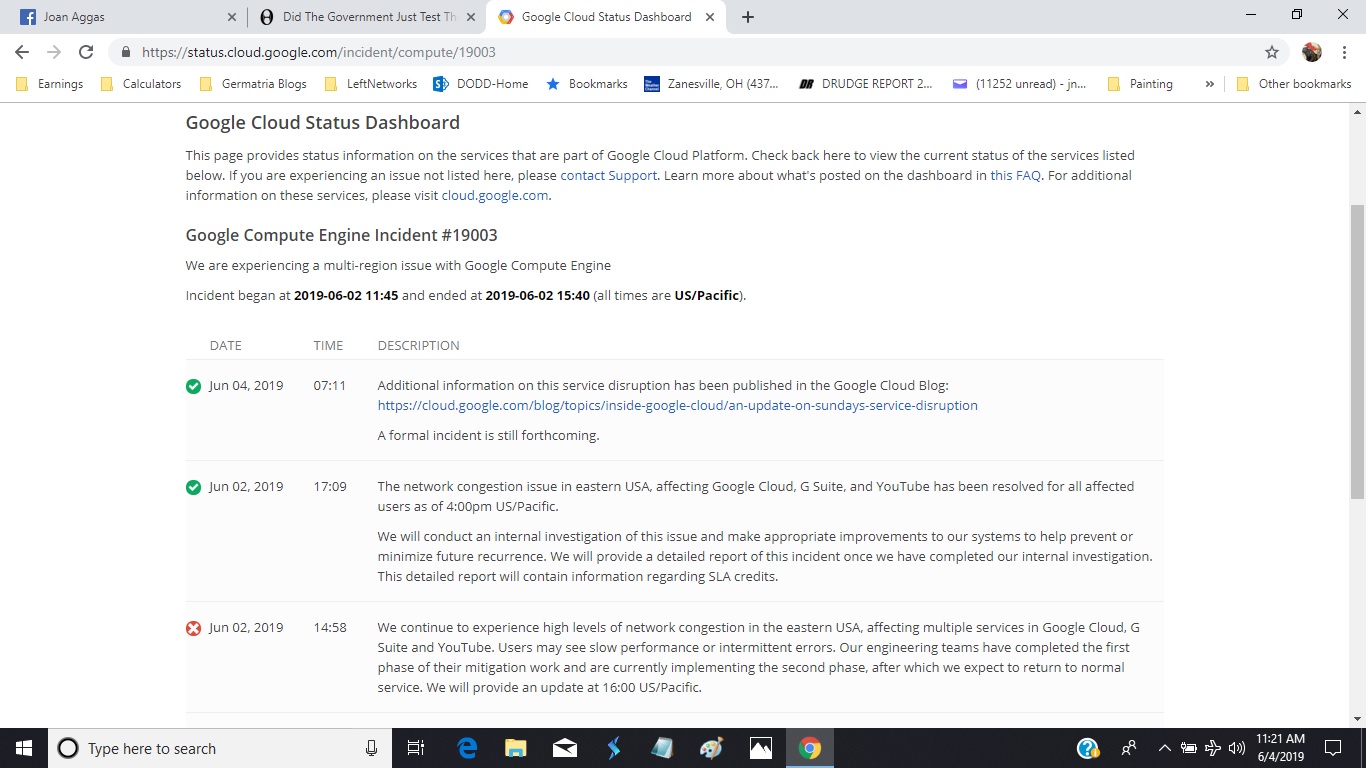The image depicts a detailed view of a computer screen displaying a web browser with three open tabs. The browser tab titles and their order from left to right are:

1. "Joan Agas" (J-O-A-N-A-G-G-A-S)
2. A partially visible tab titled "Did the government just test TH..." 
3. The selected tab, which is titled "Google Cloud Status Dashboard."

The browser's address bar shows the URL: `https://status.cloud.google.com/incident/compute/19003`. Standard browser icons are positioned to the left and right of the search bar. Below the address bar, the bookmarks bar contains various bookmarks, organized from left to right as follows:

- A folder named "Earnings"
- "Calculations"
- "Geometry Blogs"
- "Left Networks"
- "Dodd-home"
- A star icon for bookmarks
- A weather channel icon for Zanesville, Ohio, 437...
- "Drudge Report"
- A mail icon indicating "11 to 52 unread" messages
- A folder named "Painting"
- A folder labeled "Other Bookmarks."

Directly beneath the bookmarks bar, the main content area of the page shows the interface for the "Google Cloud Status Dashboard." In dark type, it states:

"Google Cloud Status Dashboard
This page provides status information on services that are part of Google Cloud Platform. Check back here to view the current status of the services listed below. If you are experiencing an issue not listed here, please contact support. Learn more about what's posted on the dashboard in this FAQ. For additional information on these services, please visit cloud.google.com."

The phrases "contact support," "this FAQ," and "cloud.google.com" are highlighted in blue.

Further down, it notes:
 
"Google Compute Engine Incident 19003
We are experiencing a multi-region issue with Google Compute Engine. Incident began at 2019-06-02 11:45 and ended at 2019-06-02 15:40. (All times are US Pacific)."

Below this statement, there are three columns labeled "Date," "Time," and "Description," listing three incidents:

1. **Date**: June 4, 2019 | **Time**: 07:11 | **Description**: A green check mark symbol is followed by "Additional information on this service disruption has been published on the Google Cloud blog," with a provided web address, indicating that a formal incident report is forthcoming.

2. **Date**: June 2, 2019 | **Time**: 17:09 | **Description**: A green check mark symbol is followed by "This network congestion issue in Eastern USA affecting Google Cloud, G Suite, and YouTube has been resolved for all affected users as of 4 p.m. US Pacific. We will conduct an internal investigation of this issue and make appropriate improvements to our systems to help prevent or minimize future recurrence. A detailed report of this incident will be provided once the internal investigation is completed, including information regarding SLA credits."

3. **Date**: June 2, 2019 | **Time**: 14:58 | **Description**: A red X symbol is followed by "We continue to experience high levels of network congestion in the Eastern U.S., affecting multiple services in Google Cloud, G Suite, and YouTube. Users may see slow performance or intermittent errors. Our engineering teams have completed the first phase of their mitigation work and are currently implementing the second phase, after which we expect to return to normal service. We will provide an update at 16:00 US Pacific."

The bottom part of the screen holds the customary status bar and icon choices typical of a Windows operating system.